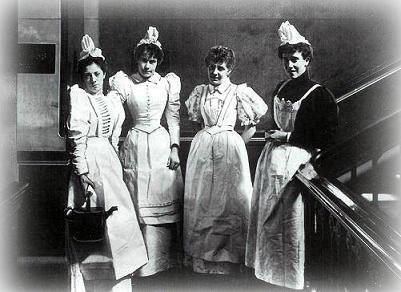In this vintage black-and-white photograph, four women stand near a staircase in what appears to be a formal, possibly professional setting. The central figure, an older woman dressed in a more expensive white gown, is flanked by three younger women. Two of these women are wearing white gowns and aprons, while the woman on the far right wears a black top beneath her apron, suggesting she is a maid. Three of the women sport hats adorned with small flowers. The leftmost woman, holding a black kettle, stands beside what seems to be a kitchen area, with a door visible to the left. They all stand in a composed pose, possibly on a floor landing, against a background of grey, capturing a distinctly vintage style.